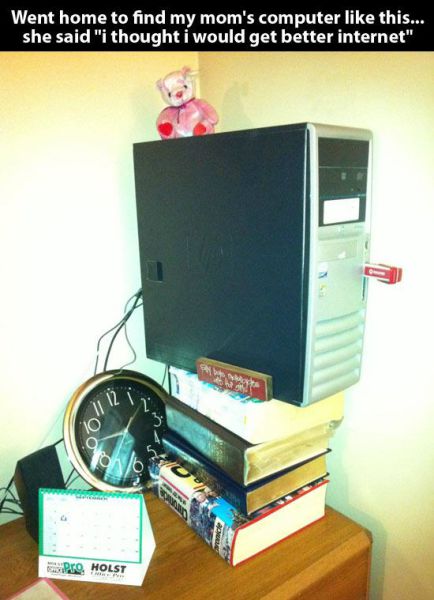The image captures a humorously cluttered home office or bedroom desk setup, with a brown desk or dresser in the bottom left corner. On the desk, there is a desktop computer case positioned diagonally atop a stack of about four thick hardcover books. Above the computer case sits a plush pink teddy bear with red hearts on its paws. Behind the stack of books, you can see a clock and a green and white calendar. A black speaker is also present on the desk, along with several cluttered objects, contributing to an overall messy appearance. The front of the computer case is gray, and some wires trail out from its back. The text, reading "Went home to find my mom's computer like this. She said, 'I thought I would get better internet,'" is placed in a black rectangle with white letters at the very top of the image, adding a humorous context to the scene. The color palette includes black, white, pink, red, gray, gold, blue, and green.